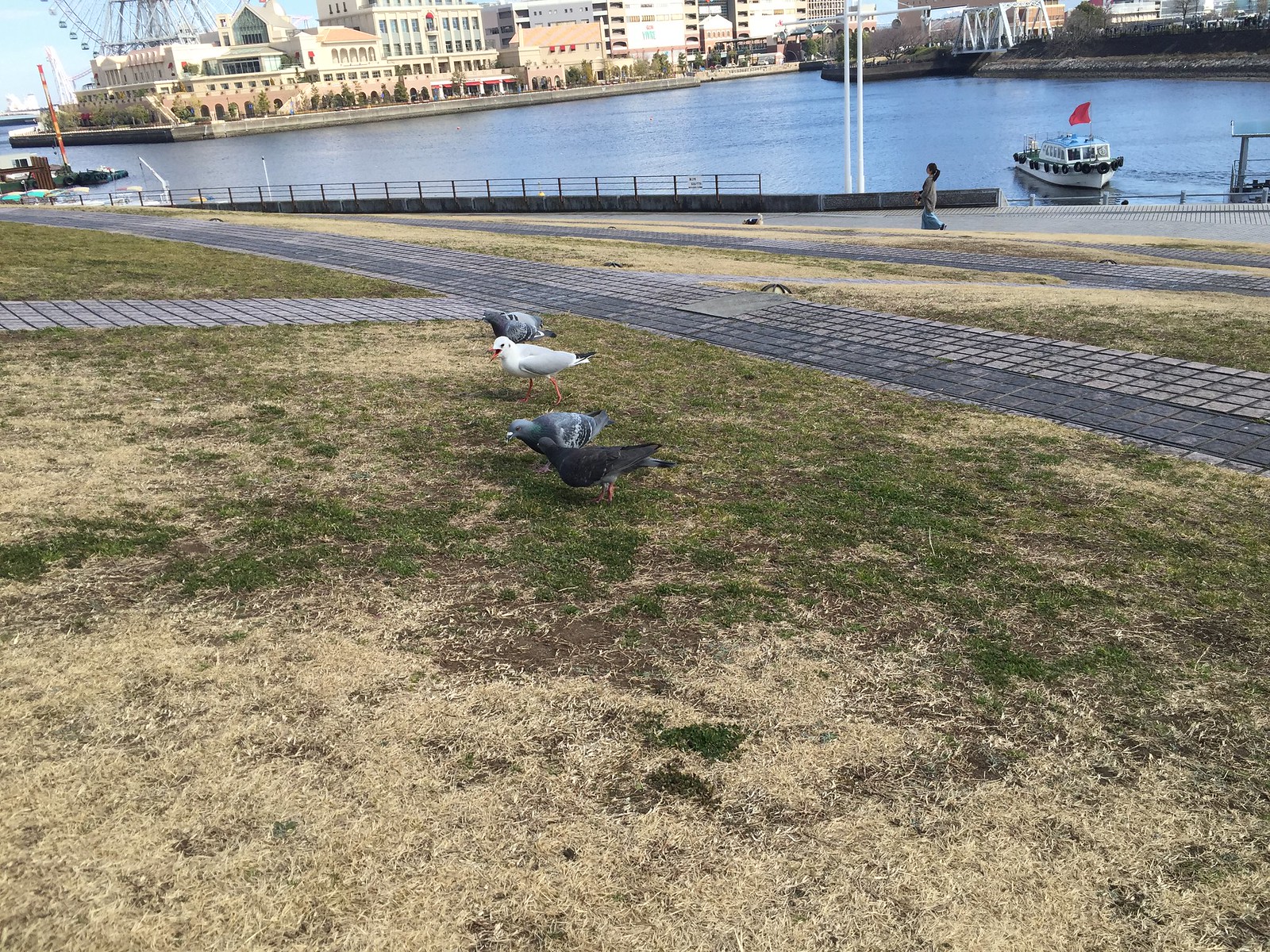This color photograph captures a lively scene near a marina or coastal area. In the foreground, three grey pigeons with spots and a distinctive white duck are pecking around a sparse, dried-up patch of grass, revealing brown soil beneath. The backdrop reveals a large river or possibly an ocean bay, stretching from the top right to the top left of the image. A small boat with a red flag on a pole can be seen to the top right, near the water's edge. There are buildings and a carousel visible across the shore, along with a person walking in the background, indicating a bustling, active area. The weather suggests it might be fall, with part of the grass looking dead and dried. The water looks light blue and the overall scene, with its busy, vibrant atmosphere, points to a picturesque but possibly cool day by the water.